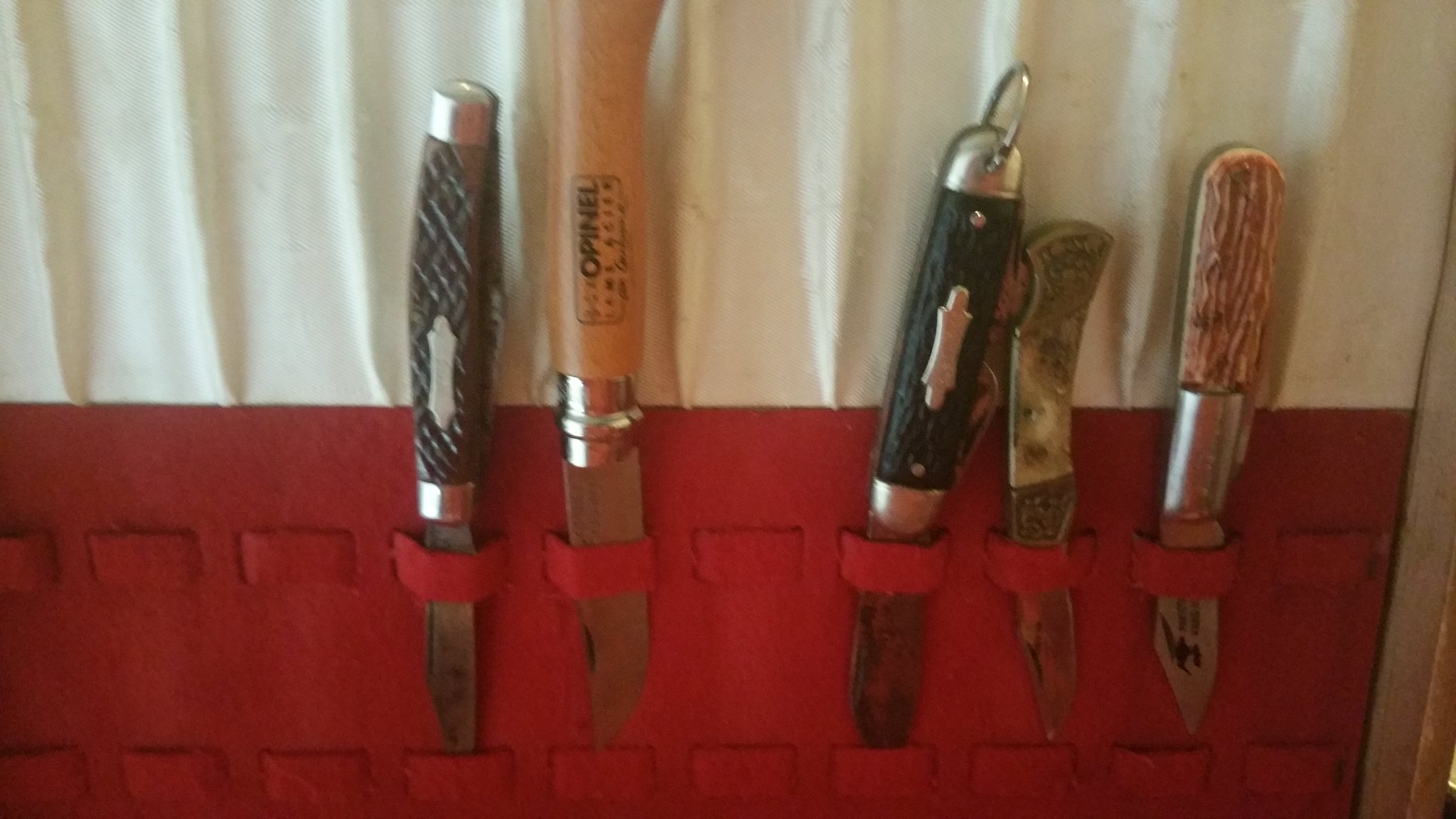The image is a close-up photograph showcasing five distinct pocket knives displayed in a knife rack. The rack is crafted from a thick red fabric, featuring multiple rows of loops that securely hold the knives. Each knife is positioned in an open state with the blades facing downward within these loops. The setup is set against a white, curtain-like background, possibly part of the case for storing the knives.

Detailed observations reveal the following about the knives: one of them resembles a switchblade with a black handle complemented by silvery metal trim. Another features an old-fashioned wooden handle. There's also a light brown, newer-looking handle inscribed with the brand name "Opinel." Additionally, there is a knife with a striking gold handle. Among the knives, several empty slots are noticeable, hinting at a neatly organized yet incomplete collection.